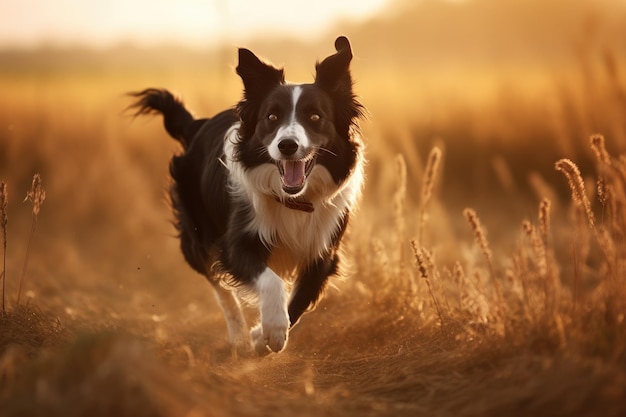In this digitally enhanced, full-color photograph taken in natural daytime light, a spirited black and white dog, possibly an English Setter or sheepdog, is captured mid-stride as it runs joyfully through a field of tan, possibly pussy willow or wheat plants. The horizontally rectangular image is rich in detail, with blurred brown and tan plants creating a sense of motion in the background. The dog's ears are flopping over its head, and its mouth is open wide with its tongue out, giving an impression of exuberant joy. Its distinctive markings include a white stripe down its black face, white above the nose, white neck, and white paws, with a black tail trailing behind. The sky, a grayish white, peeks through the upper left corner, contrasting softly with the field. The overall scene emphasizes the dog's dynamic movement, with one white paw lifted and the others in various stages of gallop, conveying vibrant energy and happiness.